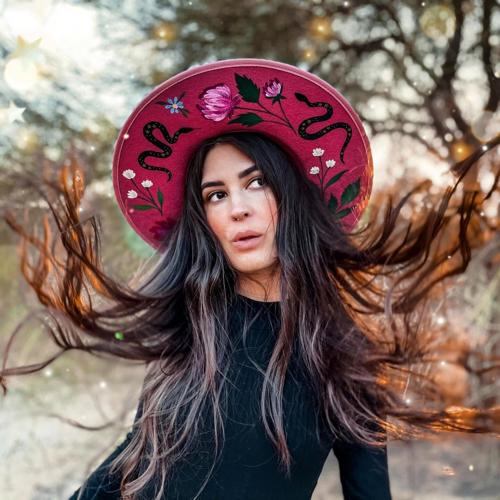This square photo captures a dramatic and elegant scene of a woman from the waist up. She is wearing a large, round-rimmed hat, predominantly dark pink or red, accentuated with a rose-colored border. The underside of the hat showcases intricate patterns including black snake images, along with pink and blue flowers with black leaves. Her long, dark brown, almost black hair flows freely in all directions, suggesting the presence of a strong breeze or a meticulously staged shot. She is adorned in a tight-fitting, long-sleeved black sweater, emphasizing her slender figure. Her face, framed by dark eyebrows and intense eyes, is turned slightly to her left, or our right, with her mouth parted subtly, adding to the mysterious allure. The blurry background features tree branches with green leaves and a cloudy sky, punctuated with dots of yellow and white light, possibly resembling fireflies or added effects. Small patches of grass and sandy ground can also be discerned, further grounding this ethereal outdoor setting.